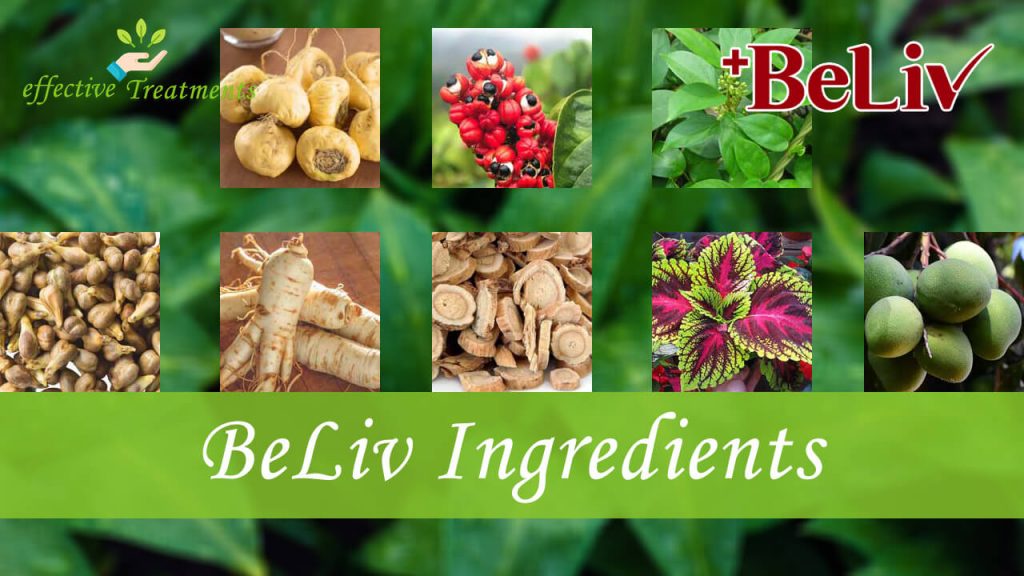The image is a horizontally oriented advertisement for "Beliv Ingredients" featuring various plants and roots. The background is a blurred green foliage with large leaves, providing a natural backdrop. There are eight inset photos, showcasing a variety of plants and fruits in vibrant colors—purple, light purple, green, red, and brown. 

In the upper left corner, there's a logo of a hand holding three leaves, accompanied by the text "effective treatments" in green letters. The text partially overlaps with the first image, which displays a bundle of light-colored roots resembling turnips. Next to it, in the center top, is a photo of red berries with contrasting black and white accents, and to the right is an image of green leaves. Positioned prominently in the top right corner is a plus sign and the word "B-E-L-I-V" in red letters. 

Below the top row of images are five more photos, featuring a mix of roots and plants. Along the bottom of the image, a green banner with white text reads "Beliv Ingredients," reinforcing the promotional message of the advertisement.